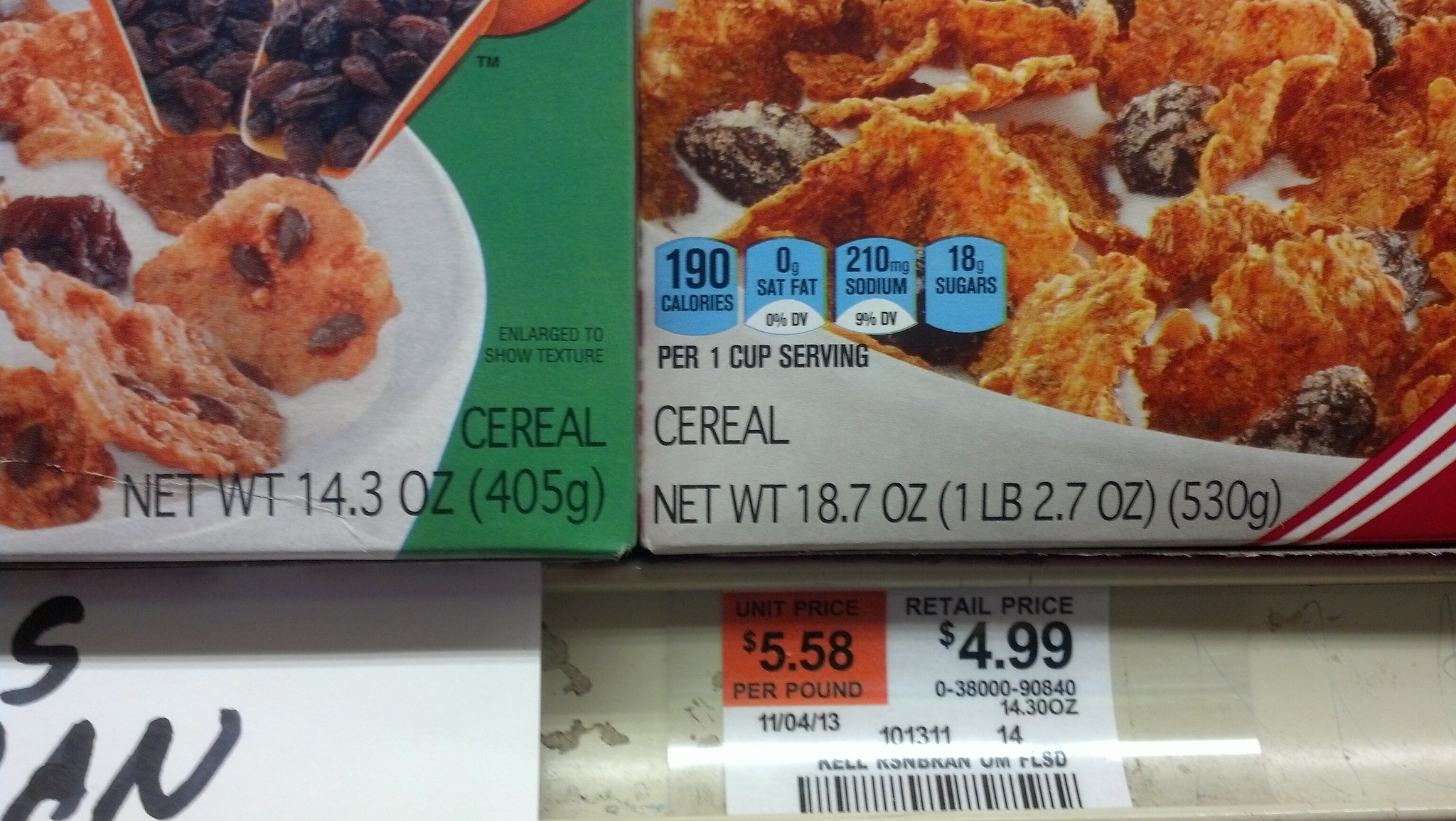This is a zoomed-in image of a grocery store shelf displaying two cereal boxes and a detailed price tag. The top half of the image shows the lower portions of two cereal boxes, each labeled 'cereal.' The box on the left features toast-like pieces with chocolate chips or possibly raisins, weighing 14.3 ounces. The cereal box on the right contains flakes with small, brown pieces, potentially raisins, and has a net weight of 18.7 ounces. The price tag beneath these boxes on the shelf is prominently in view: it lists the retail price as $4.99, the unit price as $5.58 per pound, and an additional detail of 14.30 ounces. The tag also includes a barcode and the date "11-4-13." The bottom edge of another sign is just visible on the left side of the tag, though it is partially obscured.